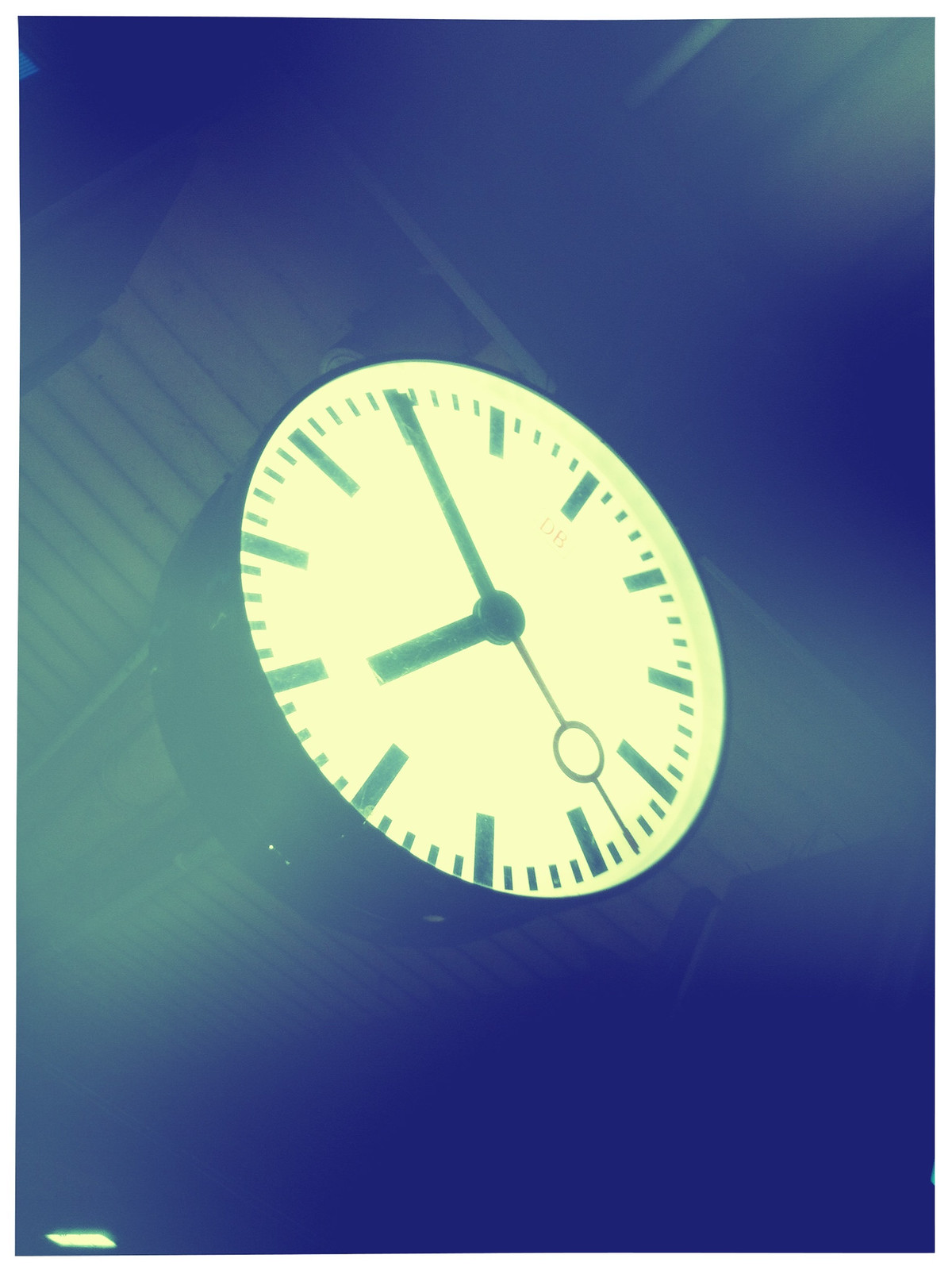This impressionistic image features a blurry clock face, as if shrouded in a fog. The background gradient transitions from black to blue, interspersed with patches of yellowish-green, creating an abstract and ethereal atmosphere. The clock face is strikingly white and circular, standing out against the moody backdrop. Instead of traditional numbers, the clock features bold black hash marks indicating the hours, with finer lines marking the minutes. The clock hands are simple and black, contrasting sharply with the white face, while a slender second hand, possibly metallic or gold, adds an elegant touch with its small oblong circle at the center. The overall composition evokes a mysterious and dreamy quality, making one question the nature of time and perception.